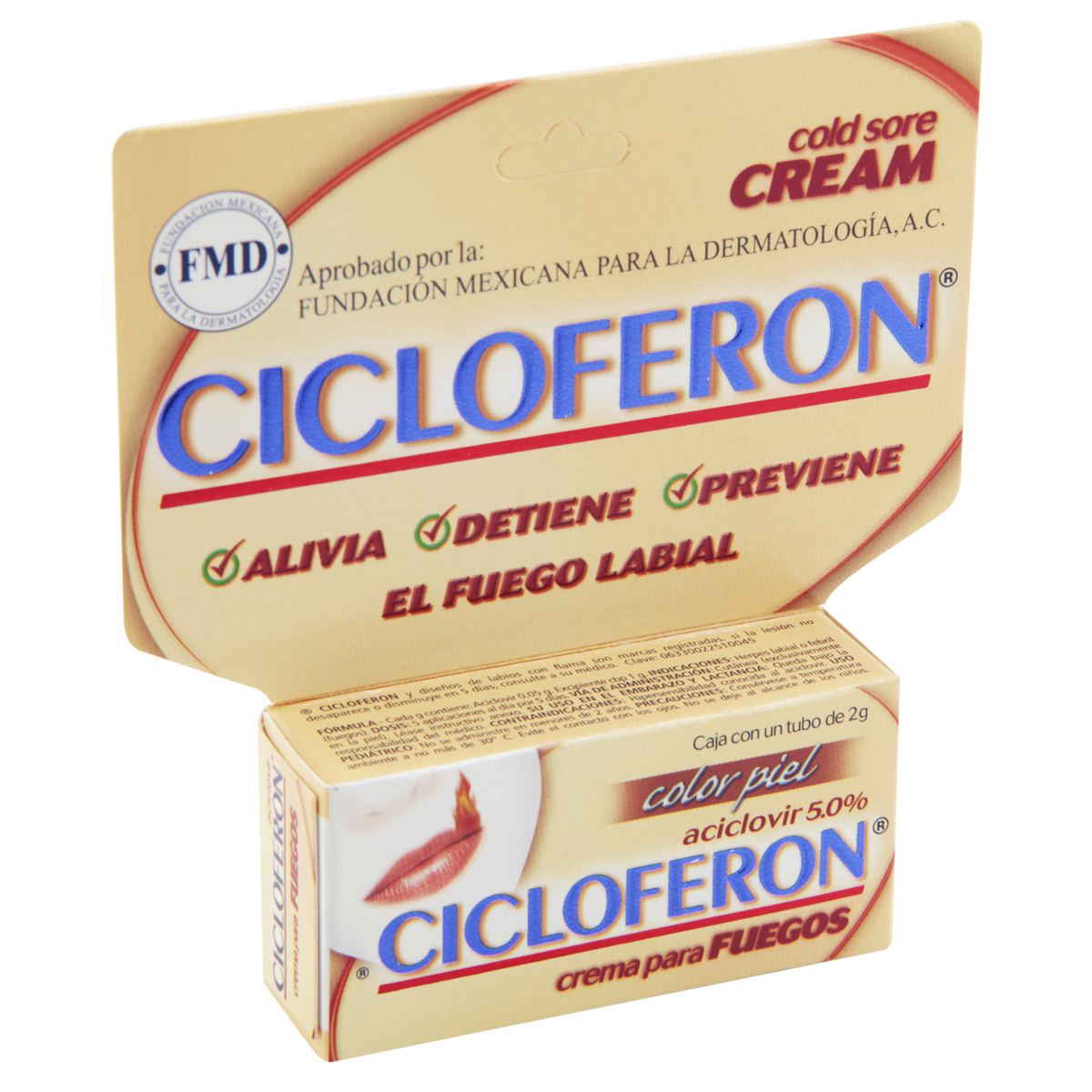This is a product image of Cold Sore Cream called Cicloferrin. The packaging is primarily a light beige or tan color with red and blue accents. "Cicloferrin" is prominently displayed in a bright blue font, underlined with a red line. Most of the other text on the box is in Spanish, with "alivia, detiene, previene, el fuego labial" written in red font, each word accompanied by a green circle with a check mark. The packaging highlights its benefits in Spanish, such as "crema para fuegos," with "color piel" indicating a skin-colored cream. Additionally, there's an image of a fair-skinned person with pink lips, showing a small red and orange flame at the left corner of their mouth. The overall design includes a white background with a tan color scheme, red lines, and some artistic elements, including a seal marked "FMD" in a white circle with dark blue letters on the top left. This package is designed for display in drugstores, featuring a standard rectangular shape with a larger display area.